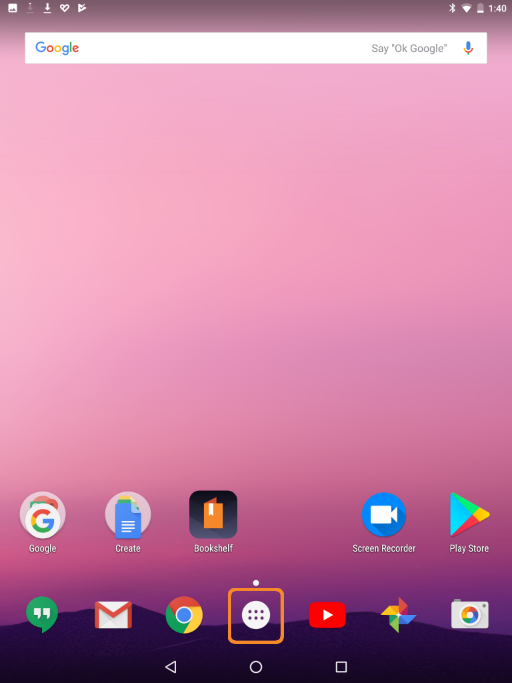This image is a screenshot of a tablet wallpaper with a wide aspect ratio. The wallpaper features a gradient background shifting from purple at the bottom to a lighter hue at the top, overlaid by the silhouette of distant hilltops. Dominating the upper portion of the screen is a large, rectangular Google search bar, adorned with the colorful Google logo on the left. To the far right of the search bar are the words "Say, 'OK Google'" in small gray print, followed by a microphone icon.

At the bottom of the screen, there are two rows of app icons. The first row begins with the Google app icon, followed by a "create" icon, and a "bookshelf" icon. There is a blank space in this row, which is then followed by the screen recorder icon and the Play Store icon. The second row contains icons for Google Hangouts, Gmail, Chrome, and an app drawer button, which is a yellow circle with six white dots in its center. Notably, an orange box has been edited onto the screenshot, obscuring the app drawer button.